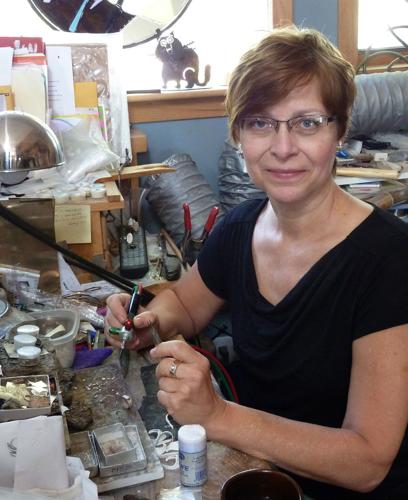In this detailed indoor photograph, a middle-aged woman is prominently featured, seated at a cluttered worktable, possibly in her workshop or a crafts shop. She has short brown hair, blue eyes, and wears glasses along with a black shirt. The woman holds a multipurpose pen, presumably used for dispensing or painting, featuring red and green cartridges. She is giving a soft, timid smile while looking directly at the camera. The table she leans on is strewn with various art materials, including several white cylindrical containers filled with glitter, along with a bottle topped with a white cap. The background reveals a vibrant space filled with numerous tools, canvases, gray tubes, and other artistic paraphernalia, contributing to an organized chaos. Two windows allow natural light to pour into the room, which has blue walls with green wood grain frames, and a noticeable duct runs along the wall. Additionally, a cat decoration adds a whimsical touch to the scene.